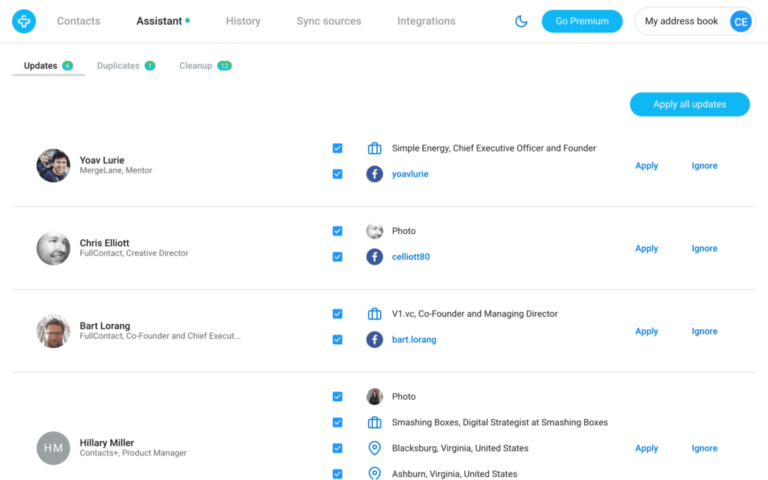**Landing Page Overview**

- **Background**: Predominantly white.
- **Top Left Corner**:
  - **Icon**: A cyan blue circle with a misshapen cross.
  - **Navigation Text**: 
    - "Context" in grey.
    - "System" in bold black with a small teal dot next to it, indicating selection.
    - "History" in grey.
    - "Sync Sources and Integrations".
  - **Half Crescent Moon Icon**: Blue.
  - **Buttons**: 
    - "Get Premium" in cyan blue with white text, oval shape.
    - "My Address Book" in an oval white button with black text.
    - "Apply All Updates" in a cyan blue oval button with thin white text, located far right.

**Left Panel**:
  - **Section Titles**:
    - "Updates" in bold black with a grey underline indicating it is selected, accompanied by a dark green circle with an unrecognizable symbol.
    - "Duplicates" with a green circle bearing a white line and the number 1.
    - "Clean Up" showing the number 12.

**Profiles**:
  1. **Yoav Lurie**:
     - **Photo**: Light-skinned individual with a child behind him, both wearing blue, short round hair.
     - **Name**: Yoav Lurie in bold black.
     - **Details**: "Merge Lane Mentor".
     - **Options**: Two dark blue squares with white check marks indicating selection.
     - **Buttons**: Cyan blue oval button with white "Apply All Updates" text.
     - **Additional Info**: 
       - Position: Chief Executive Officer and Founder of Simple Energy.
       - Facebook: Yoav Lurie (hyperlink in cyan blue).
       - "Apply" and "Ignore" buttons.

  2. **Chris Elliott**:
     - **Photo**: Close-up, gray and black image.
     - **Name**: Chris Elliott in bold black.
     - **Details**: "Full Contract, Creative Director, Full Content Creative Director Contact" in regular grey text.
     - **Options**: Two dark blue squares with white check marks indicating selection.
     - **Facebook**: c.elliott.av (hyperlink in cyan blue).
     - **Buttons**: "Apply" and "Ignore".

  3. **Bart Lorang**:
     - **Photo**: Light-skinned, wearing glasses, beard, white curtains and walls background.
     - **Name**: Bart Lorang in bold black.
     - **Details**: "Full Contact, Co-founder and Chief Executive" (partially cut off).
     - **Position**: Co-founder and Managing Director of VIVC.
     - **Facebook**: Bart.Lorang (hyperlink in cyan blue).
     - **Buttons**: "Apply" and "Ignore".

  4. **Hilary Miller**:
     - **Photo**: Gray circle with "HM" in white.
     - **Name**: Hilary Miller in bold black.
     - **Details**: "Contacts Plus Product Manager".
     - **Position**: Digital Strategist at Smashing Boxes.
     - **Location**:
       - Blacksburg, Virginia, USA.
       - Ashburn, Virginia, USA.

Each profile's description includes visual elements, job titles, social media handles, options, and actions to be taken, providing a comprehensive overview of individuals presented on the page.